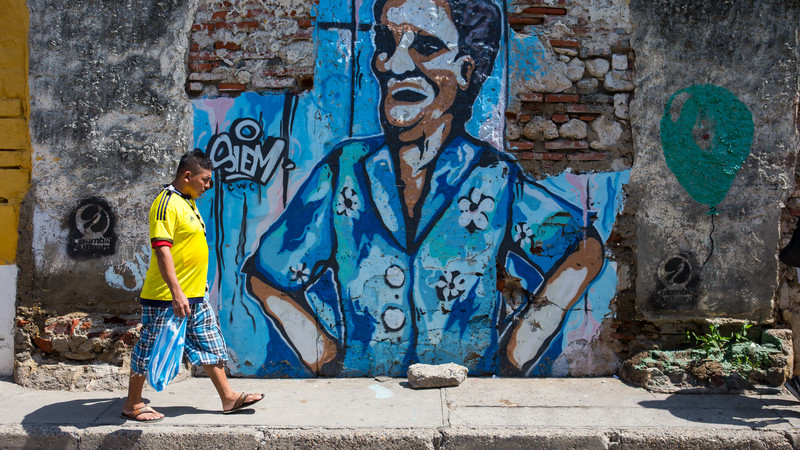This outdoor photograph captures a man walking along a sunlit sidewalk, casting a shadow behind him. Positioned on the left side of the image, the man wears a bright neon-yellow shirt adorned with black stripes on the shoulders, paired with blue and black plaid shorts, and sandals. He holds a blue plastic bag in his hand and appears to be looking down as he walks from left to right. The background features a somewhat dilapidated rock wall with vibrant graffiti artwork. Dominating the center of the image is a mural depicting a man with brown skin, wearing a blue Hawaiian shirt with white floral patterns, his elbows bent with hands on hips, and his mouth open, creating an impression of judgment or laughter toward the passerby. The graffiti includes bright blue and tan hues for skin tone. To the left of the mural, the letters "O-I-E-M" are spray-painted graffiti-style, and to the right, a green balloon is painted above a segment of the brick wall. The surrounding context of the location remains unidentified.